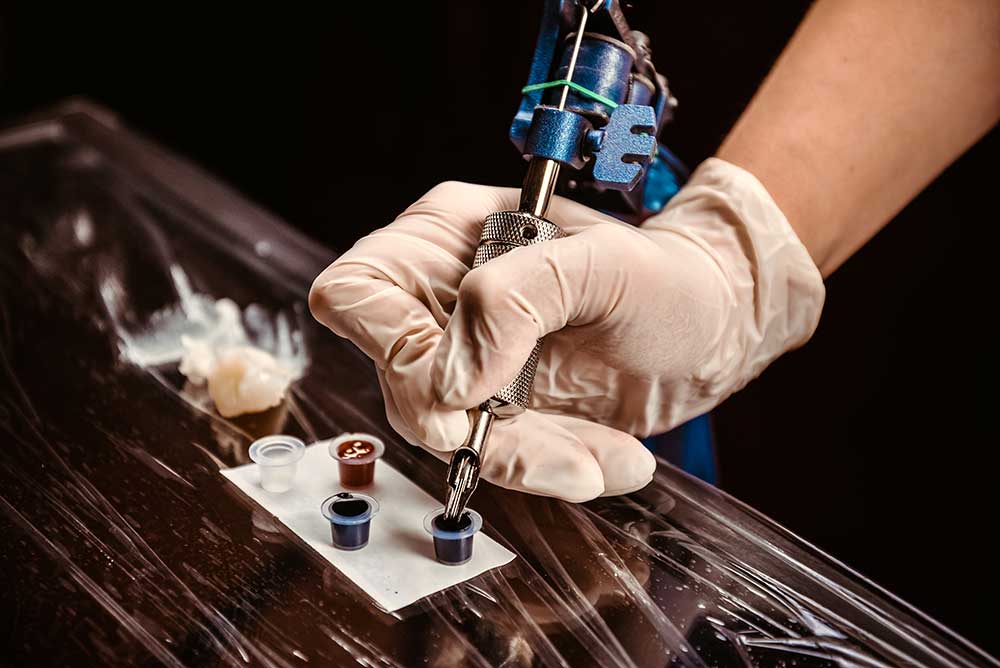This detailed, close-up photograph showcases a tattoo artist's gloved hand, adorned in a white latex glove, as they intricately dip a mechanical tattoo needle into a small, plastic container of dark black ink. The tattoo machine itself is a striking blend of blue and silver stainless steel, featuring a distinctive green band around the top. The scene unfolds atop a table covered in a protective plastic sheet, secured by a white piece of paper, ensuring a hygienic workspace typical of a tattoo shop environment. Surrounding the black ink are additional tiny ink wells containing red and blue pigments, along with a jelly-like substance set upon the plastic covering. The deeply dark and blurred background contrasts sharply, drawing the viewer's attention entirely to the precise moment of ink application.